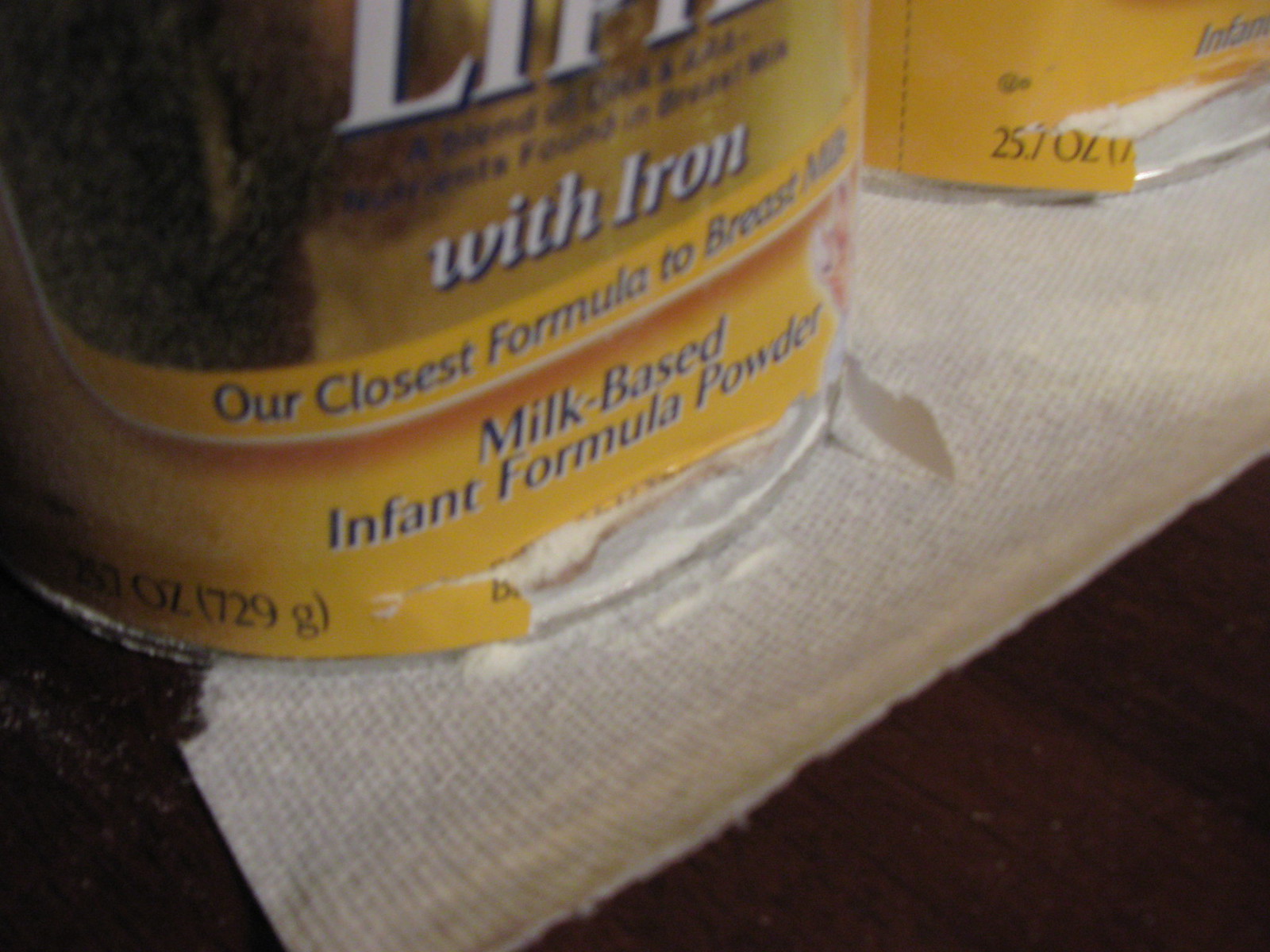Here's a detailed and cleaned-up caption for the image:

---

This image provides a close-up view of a damaged can of infant formula. The front bottom edge of the gold can is ruptured, causing formula to spill onto a section of white paper towel. The top part of the photo shows a partial view of the brand name containing the letters "life," followed by out-of-focus black text. Prominently displayed in large white letters is the phrase "with iron," beneath which a yellow banner reads, "our closest formula to breast milk." Below this banner, it states, "milk-based infant formula powder." The label on the left and right sides is torn, exposing the silver bottom of the can, which is scattered with formula powder.

Adjacent to this can, positioned in the top right corner, is the edge of another can with a similar issue — it too is busted at the bottom. Both damaged cans rest on a white paper towel, which is placed on a brown wooden table.